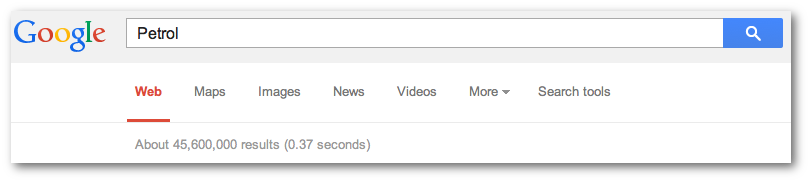This image is a screenshot from a tablet, depicting a Google search page. In the upper left corner of the screen, the Google logo is prominently displayed. The logo's letters are brightly colored in the following sequence: the first "G" in blue, the first "O" in red, the second "O" in yellow, the second "G" in blue, the "L" in green, and the "E" in red.

Beneath the logo, there is a long rectangular search bar. Inside this bar, the search term "PETROL" is typed in capital letters. To the right of the search term, there is a blue search button featuring a magnifying glass icon.

Directly below the search bar, a navigation menu is present. The first option, "Web," is highlighted in red with an underscore. Adjacent options in light gray include "Maps," "Images," "News," and "Videos," followed by "More" and "Search tools."

Below this navigation menu, the search results are indicated. The text reads "About 45,600,000 results" with the time taken to generate these results in parentheses, stating "0.37 seconds." The background of this section is white, while the area behind the Google logo and the search bar is light gray.

Overall, the screenshot successfully captures the essence of a Google search page, with clear and vivid details of each element.